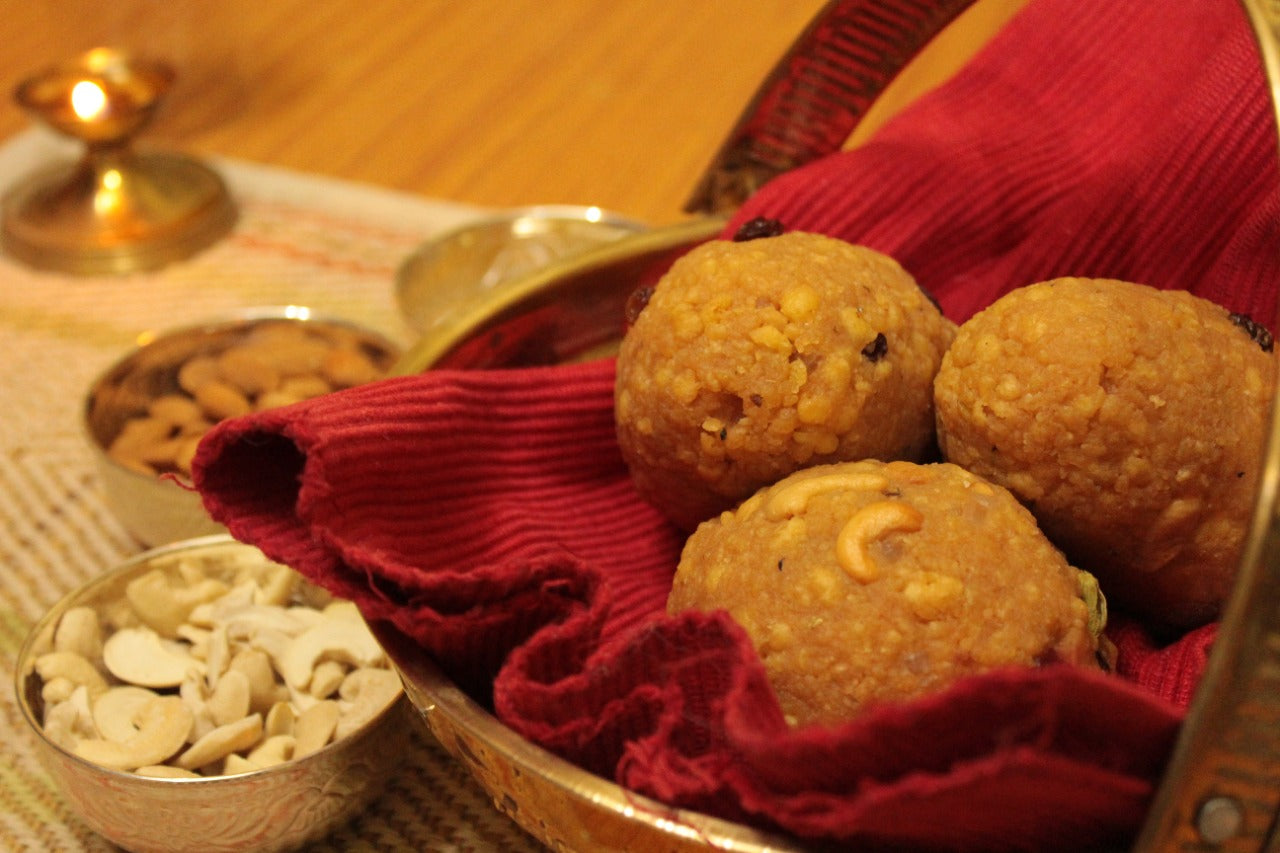This close-up photograph, likely taken inside a restaurant, features a gilded faux-golden metal basket lined with a vibrant red cloth, holding three lightly browned, grainy muffins. These muffins, speckled with visible cashew nuts, display golden-brown tops with some yellow or orangish bumps. The basket sits prominently, slightly right of center, while its handle arcs elegantly out of the frame's upper right and left edges. Adjacent to the basket on a plaid tablecloth lie three smaller metal bowls, containing various nuts. The top bowl holds almonds, the middle one's contents are indiscernible, and the bottommost bowl is filled with cashews. The wooden dining table's surface peeks through at the top of the image, along with a small golden object, possibly a goblet or candle holder, lending a touch of mystery to the setting.